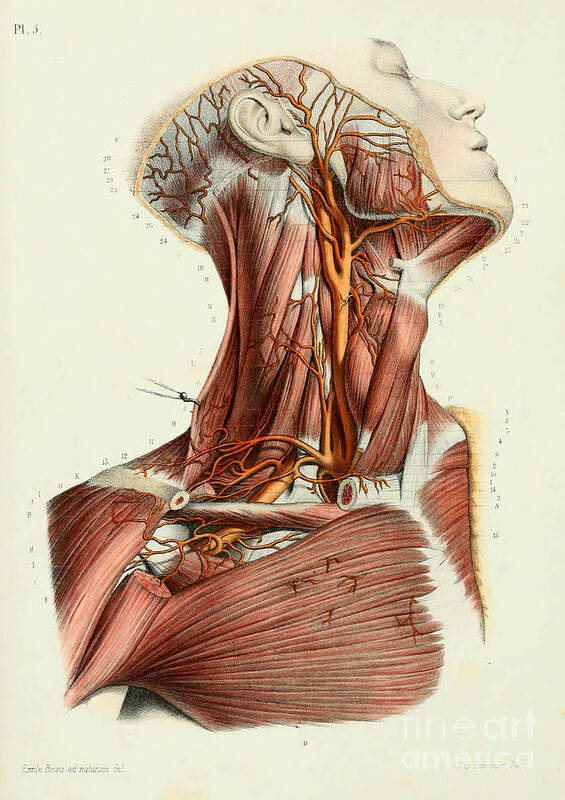This image is a detailed anatomical drawing from an old medical book, representing a person in a side view. The individual's head is tilted back and facing upwards to the right, revealing intricate details of the neck and upper torso muscles. Their face, ear, nose, mouth, and one eye are sketched in pencil, while the rest of the body is depicted in a cutaway view with the skin removed to expose the underlying red muscles and orange veins. The fibrous muscles in the neck and the upper chest, particularly the strained muscles and arteries, are prominently shown.

The background of the image is a beige or ivory color, adding to its vintage appearance. Small numbers and hooks are scattered around the drawing, aiming to label different anatomical parts, although they appear faded and hard to read due to the aged paper. In the upper left corner, the notation "PI3" is visible, while the lower left corner contains small, faded text that reads "Emil Bau Ad Naturum Del." Additionally, there is a white watermark in the lower right corner stating "Fine Art America." This detailed sketch serves as a classical representation of the human muscular and vascular systems for educational purposes.